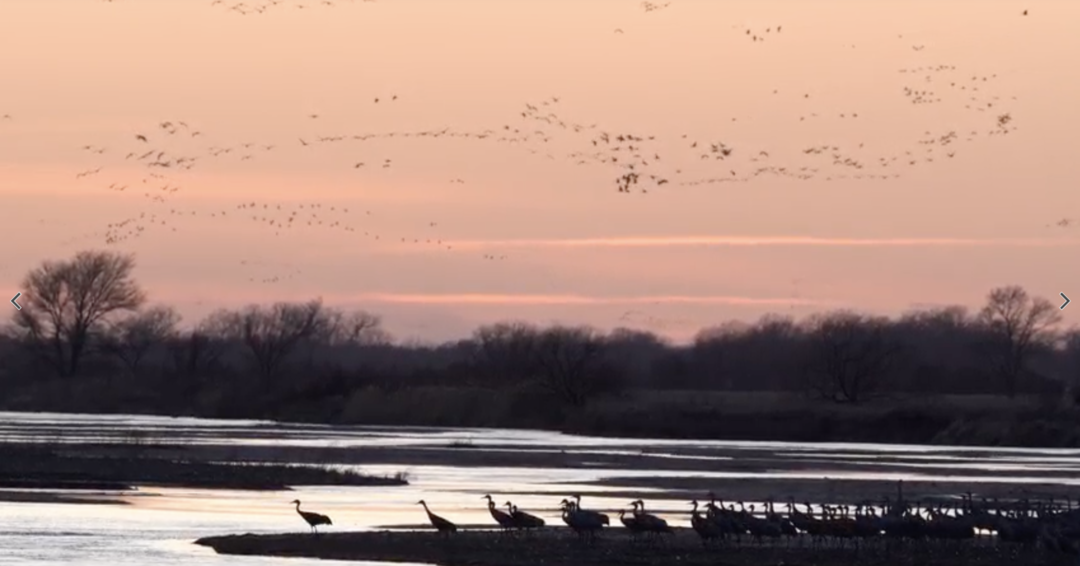This outdoor color photograph, taken at either dusk or early dawn, captures a serene and shadowy wildlife scene by a large body of water. The sky above is a beautiful blend of orange, pink, and white hues, with clouds that enhance the ethereal atmosphere. In the foreground, silhouetted against the reflective water, a large gathering of birds, possibly geese or swans, are either preparing to take a swim or to continue their flight. The birds are depicted in various stages of motion, with some captured in low detail up in the sky, forming an extensive flock of approximately 300 to 400 individuals, and others appearing in greater, though still silhouetted, detail closer to the water. In the middle of the image, the tops of barren trees rise starkly against the colorful sky, suggesting that the season might be fall or early spring. The overall ambiance of the photograph is dark and mysterious, with the silhouettes of the birds and trees creating a striking contrast against the soft, glowing sky.